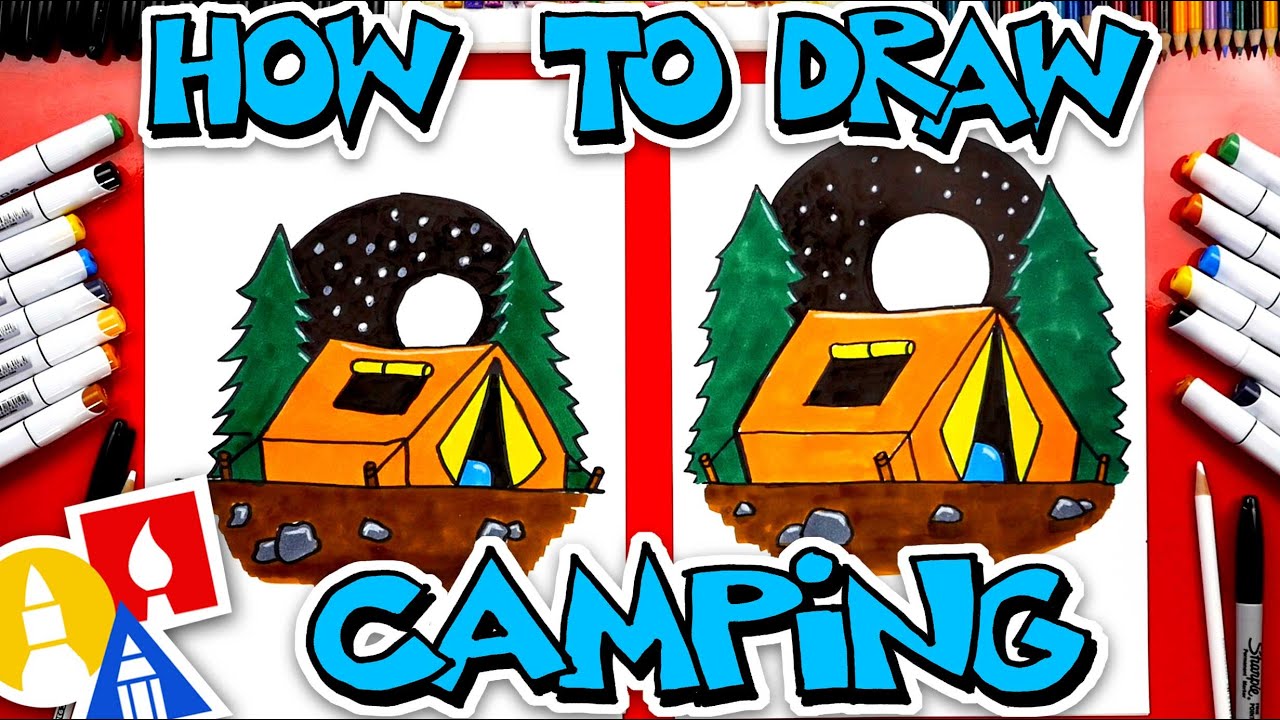The image displays an instructional "How to Draw Camping" guide, prominently titled with bold, blue capital letters outlined in black and white borders. Centered within the scene are two colorful drawings of camping setups, each featuring an orange tent with yellow doors and a rolled-up window. The tent rests on brown ground adorned with gray rocks. Flanking the tent, green trees rise against a black night sky dotted with a full white moon and bright stars. Surrounding these drawings, various markers and pens are scattered on a red table, adding to the creative atmosphere. This visually engaging image combines detailed illustrations and art supplies, making it an inviting guide for aspiring artists.